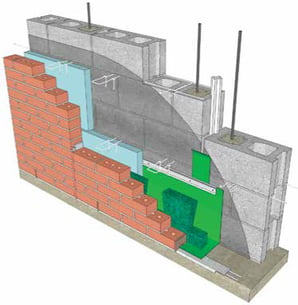The infographic is a detailed 3D cross-sectional model of a commercial building's layered wall structure. From the outermost to the innermost layer, it begins with traditional red brick-colored facing bricks. Behind the bricks is a blue layer of insulation, followed by a green vapor barrier. The innermost structural layer consists of gray concrete cinder blocks, each featuring hollow openings reinforced with metal rebar rods running vertically through them. The layers are meticulously illustrated to show each material's placement and function within the wall.